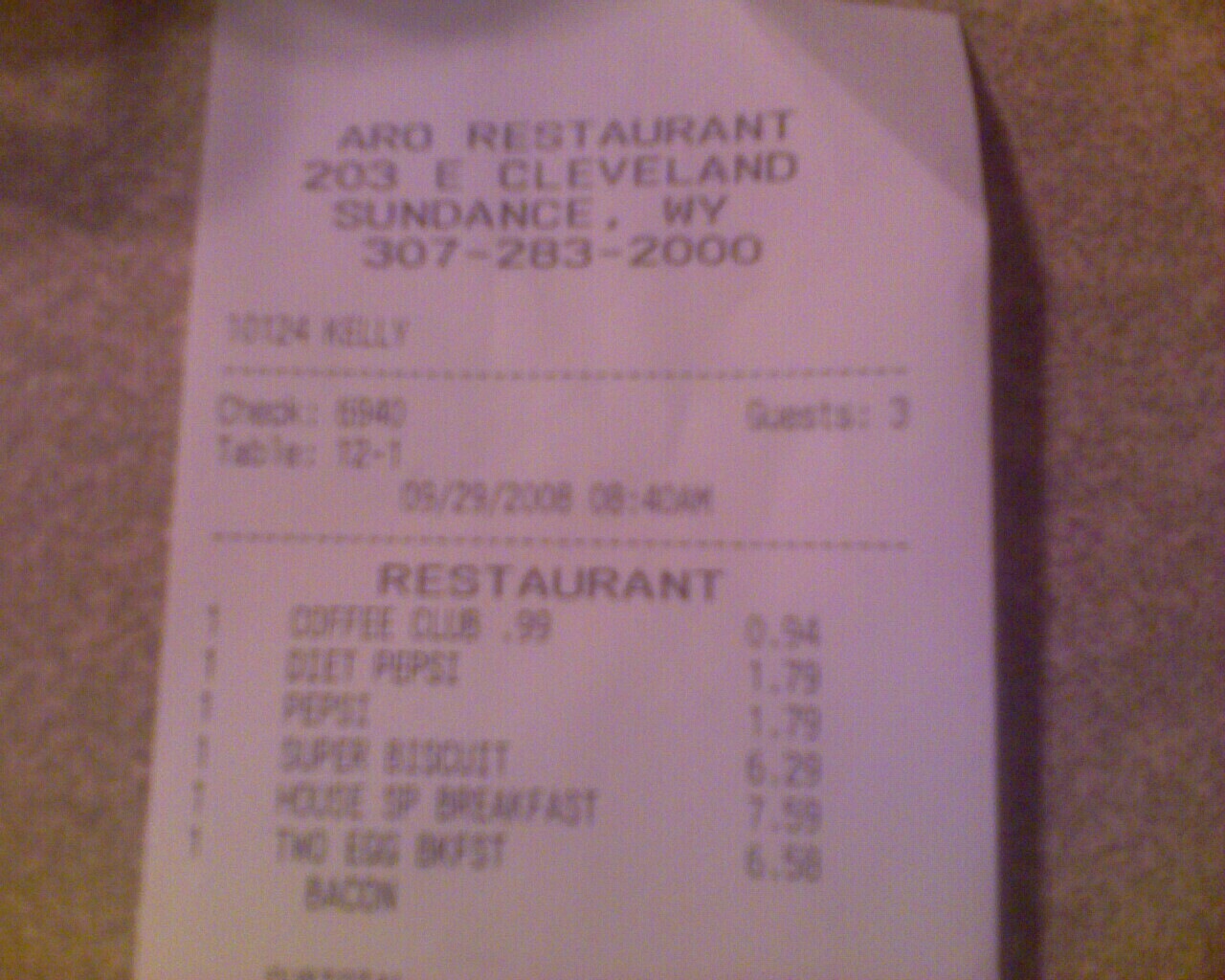In this horizontally-oriented rectangular image, we see a slightly grainy, low-resolution photograph of a restaurant receipt, placed against what appears to be a beige granite countertop. Despite the image quality, the details on the receipt are discernible. The header of the receipt reads "Aero Restaurant," located at 203 East Cleveland, Sundance, Wyoming, with a contact phone number of 307-283-2000. The order was made for three guests on September 29, 2008. The listed items include a coffee, a diet Pepsi, a Pepsi, a biscuit, a house breakfast, and a serving of two eggs with bacon.